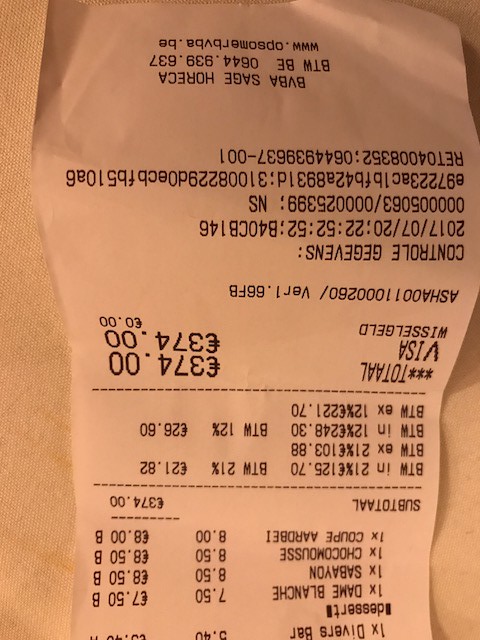This is a highly detailed photograph of a white receipt lying upside down on a tan woven or brown surface, possibly a table or mat. The receipt, printed in black ink, details a dining purchase with the printed date of 2017-07-20 at 22:52, signifying an evening transaction. Notable purchases listed include items such as "Dame Blanche" for $7.50, "Sabayon" for $8.50, "Chocolate Mousse" for $8.50, and "Coupe Aardbei" for $8.00. The subtotal amounts to 374, which could be in pounds or Euros, although the consensus leans towards it being a European currency. Payment was made using a Visa card, and additional details such as a control number and the phrase "BVBASAGE HORECA" are visible towards the bottom of the receipt.